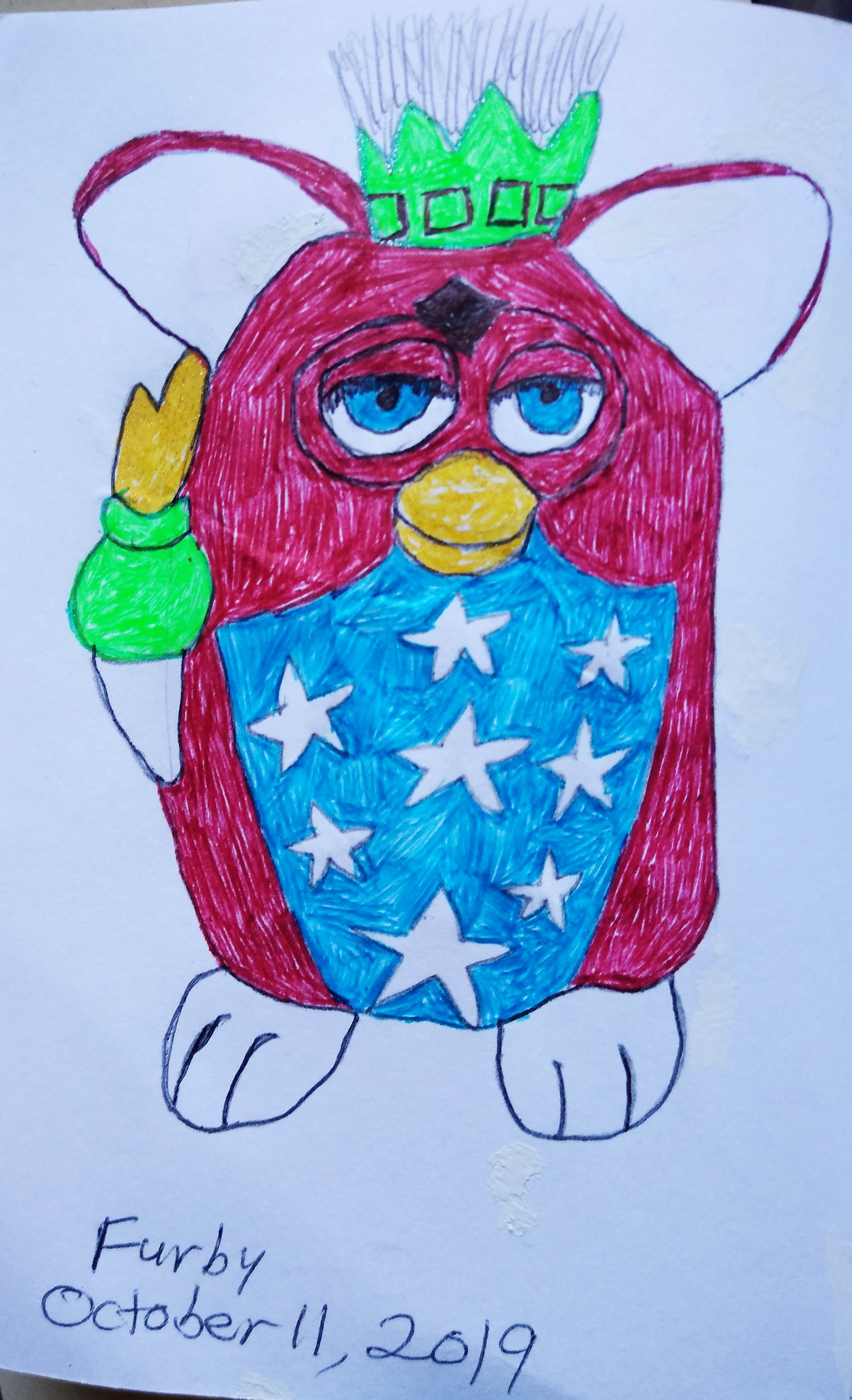This photograph captures a section of a hand-drawn illustration on a very light blue piece of paper. The lower portion of the image is slightly cropped but prominently features the text "Furby, October 11th, 2019" written in what appears to be a slightly darker blue, perhaps using pencil or magic marker. The drawing depicts a whimsical Furby character, reminiscent of the popular electronic pet from years past. This Furby stands out with its large, goofy blue eyes and a yellow beak-like mouth, both iconic features.

The body of the Furby is vividly colored in red, contrasting sharply with its floppy ears. Notably, the Furby's belly displays a patriotic theme with a star field—a blue background speckled with white stars. Atop the Furby's head sits a bright lime green crown, adding an element of regal playfulness to its appearance. The small feet are sketched simply, likely with a dark blue marker or pen. This detailed and colorful drawing captures the essence of the beloved Furby character with a creative twist.